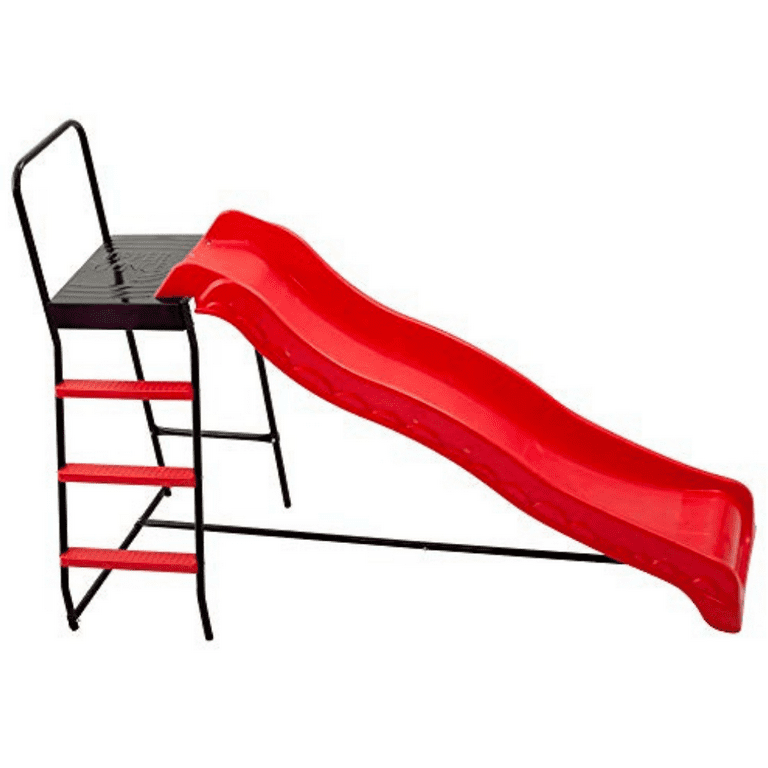This horizontal image showcases a unique children's playground slide ingeniously integrated with a chair. The slide, constructed from bright red plastic or fiberglass, is designed to be mounted on a metal chair frame. The chair itself features metal legs and supportive braces on one side, while the opposite side is equipped with three red plastic steps, allowing children to climb to the top. The chair's backrest resembles a simple railing without padding, suggesting it serves more as a structural support for the slide than a comfortable seating option. For safety, young children would need assistance ascending the steps and supervision while sliding down, as the design lacks handrails for secure grips.